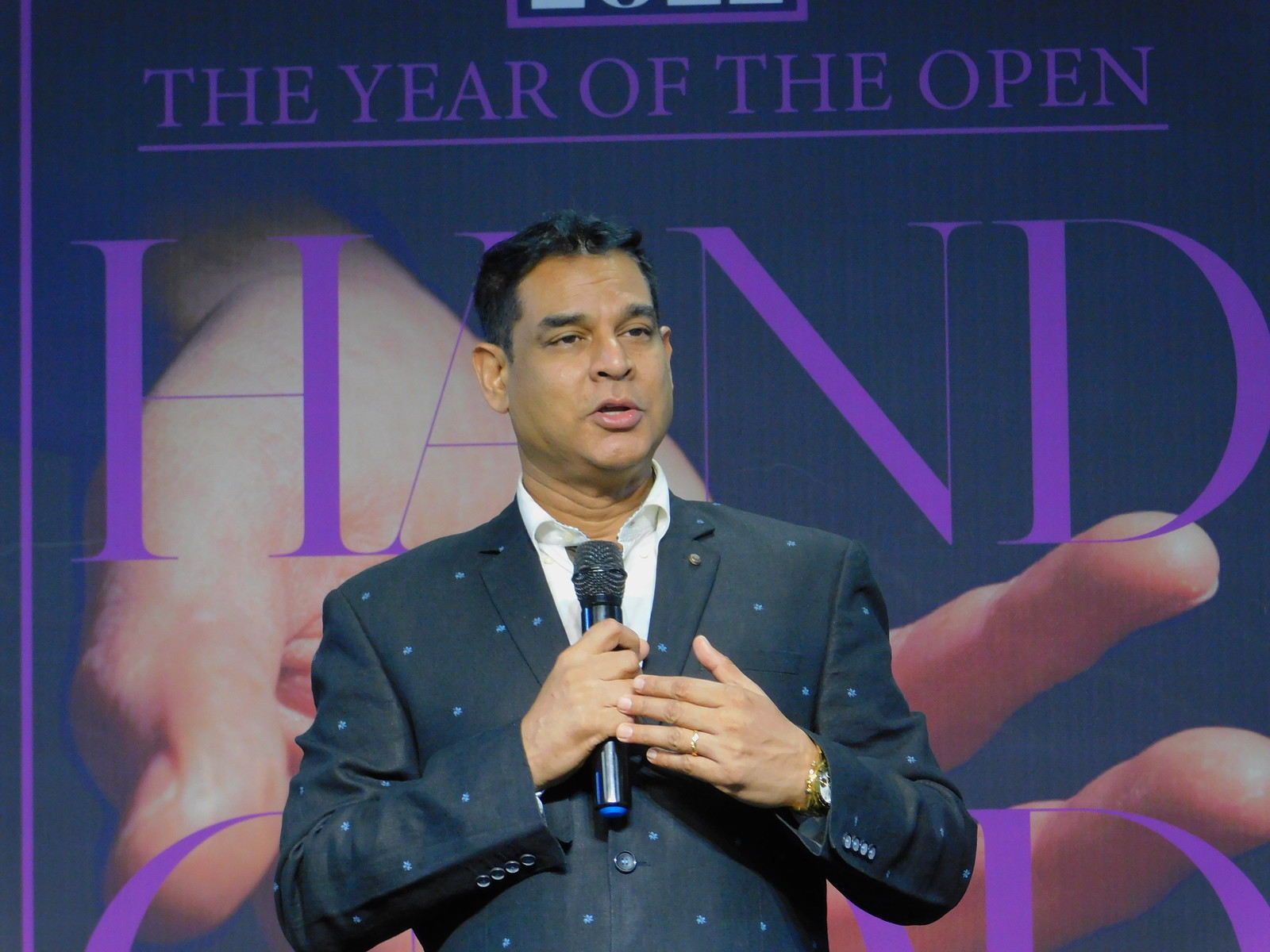This full-color photograph captures a dark-haired gentleman in his late 30s to early 40s, appearing to be of Indian descent, addressing a crowd at an event. He is wearing a dark-colored blazer adorned with light blue polka dots, paired with a white shirt but no tie. A gold wristwatch glints on his left wrist, which is also adorned with a gold wedding band. He is holding a microphone as he speaks, with his left hand touching his right. Behind him, a large poster features a blue background with the phrase "the year of the open hand" in purple and pink text. The poster includes a prominent image of an open hand reaching outward, palm up. This visual emphasizes the theme of the event as the man looks towards the right, seemingly in mid-speech.